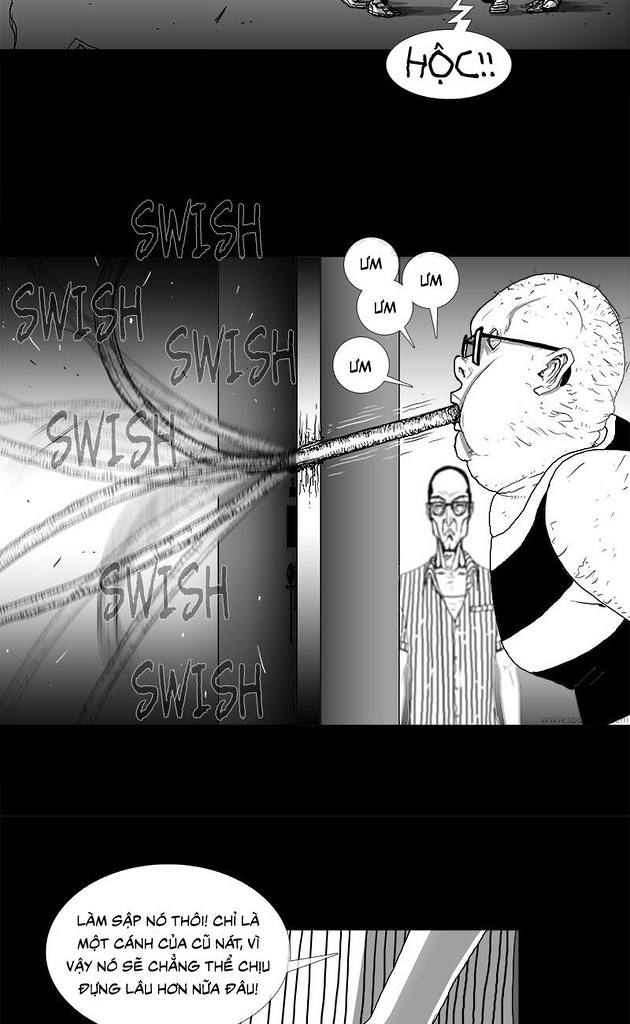This detailed black and white cartoon-style image appears to be a frame from a manga, possibly with Vietnamese text. The image is divided into two main sections, forming a rectangular layout. The upper part features a figure, potentially a man or a woman, standing slightly sideways with a long tongue or a tube extending from their mouth and twisting through the scene. This figure's dialogue bubble repeatedly says "um um um um," and the tongue/tube makes a "swish swish swish swish" noise as it moves erratically. Another man, visible only from the waist up, stands in the background; he is dressed in vertically striped pajamas or a striped shirt and wears glasses, observing the peculiar scene.

Near the top of the image, there is an additional word bubble descending from the edge, spelling out "H-O-C." The bottom of the image appears to transition to the next scene, where a dialogue bubble, written in what seems to be Vietnamese text, is visible but untranslated. A portion of the striped clothing from the man in the upper scene reappears, linking the two sections visually and thematically.